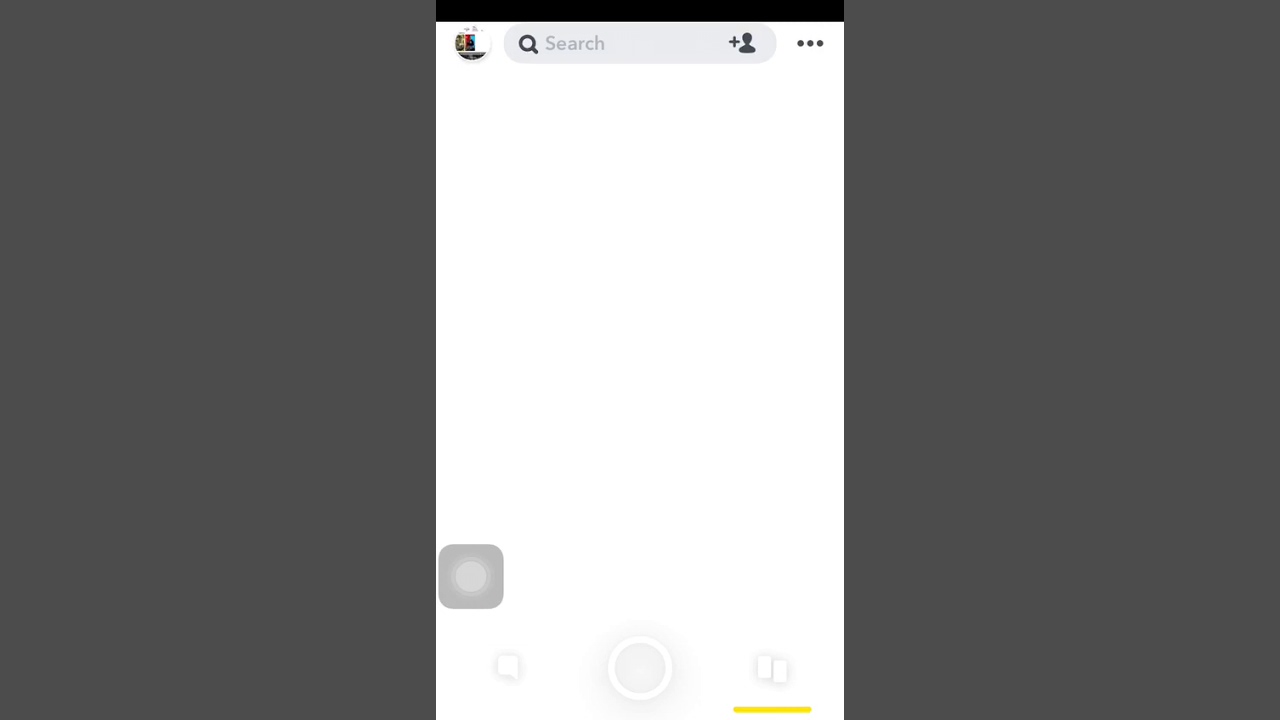The image is a detailed screenshot of a smartphone interface. The background of the screenshot is uniformly gray. 

At the top of the image, there's a black, empty banner stretching across the width of the screen. Below this banner, towards the left side, there's a circular shape. Stretching across the center of the screen is a search field, identified by a magnifying glass icon on its left side and the word "search" displayed in gray text within the field. To the far right of the search field, there's a plus icon accompanied by a user icon, followed by a set of three vertical dots indicative of additional options.

The rest of the screen below this section is predominantly white. On the lower left side, there's a gray square with a lighter gray circle centered within it. At the bottom center, a faint white circle is visible. To the right of this circle, there is an indistinct icon with a yellow line directly underneath it. This yellow line likely serves as an indicator or highlight for the corresponding icon. This detailed analysis covers the primary visual elements present in the screenshot.